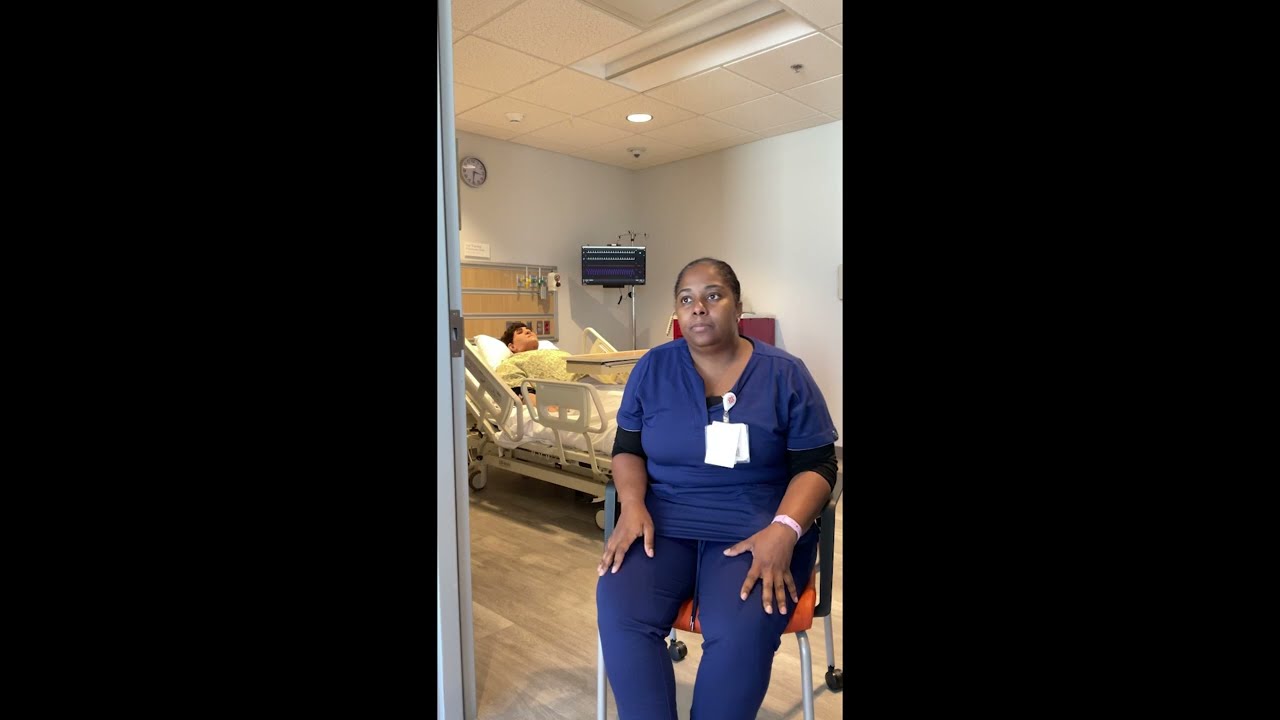In this detailed vertical-letterbox photo of a typical hospital room, an African-American woman in blue scrubs, appearing as a medical worker, is seated on an orange chair with metal legs just inside the doorway. Her ID badges are clipped to her collar, and she has a long-sleeved shirt underneath her scrubs. Her hands are outstretched in her lap, and she looks tired and somewhat worried as she gazes out of the room. The hospital environment features white walls, a tiled ceiling with bright lights, and a floor that resembles wood plank or tile. In the background, a male patient wearing a yellow hospital gown lies asleep on an inclined hospital bed with white sheets. Behind him, a monitor presumably displays vital signs, contributing to the typical clinical setting. The entire scene evokes a sense of quiet vigilance within the professional yet taxing atmosphere of the hospital.